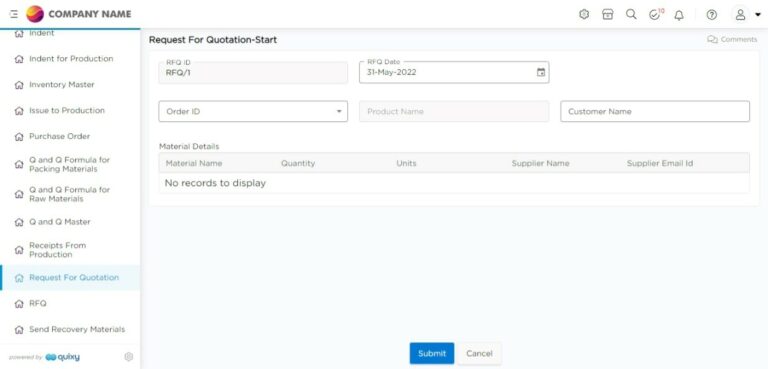**Detailed Caption:**

This image appears to be a slightly blurry screenshot of a website interface, possibly captured by a camera. On the left-hand side, there is a vertical navigation menu. At the top of the menu is a circular logo with a design that features shades of purple, yellow, and red, resembling a sun. Below this logo, the text "Company Name" is displayed.

The menu contains several options, each accompanied by an icon of a house. The options listed in descending order are: "Incident," "Indent for Production," "Inventory Master," "Issued to Production," "Purchase Order," "Q&Q Formula for Packing Materials," "Q&Q Fuel Formula for Raw Materials," "Q&Q Master," and "Receipts from Production." The currently selected option is "Request for Quotation," identified by both the highlighted section in the menu and the corresponding content displayed on the right side of the webpage.

On the main part of the webpage, the heading "Request for Quotation" is prominently displayed in black. Below this, the abbreviation "RFQ" is listed. The form includes fields such as 'RFQ ID' with "RFQ/1" already filled in, 'Date,' which is set to "31st of May 2022," and other categories like 'Order DS,' 'Product Name,' and 'Customer Name.' Some of these fields are editable while others are grayed out. Additional fields are also visible but not labeled in the provided description.

At the bottom of the form, there are buttons labeled "Submit" in blue and "Cancel" in white.

In the top-right corner of the webpage, several icons line up horizontally: a profile icon (a person silhouette), a question mark, a bell, a checkmark, a magnifying glass, a house icon, and a cogwheel (likely for settings).

At the bottom of the left sidebar, a tagline reads "Powered by QuickSee," accompanied by a blue logo and another icon to the right.